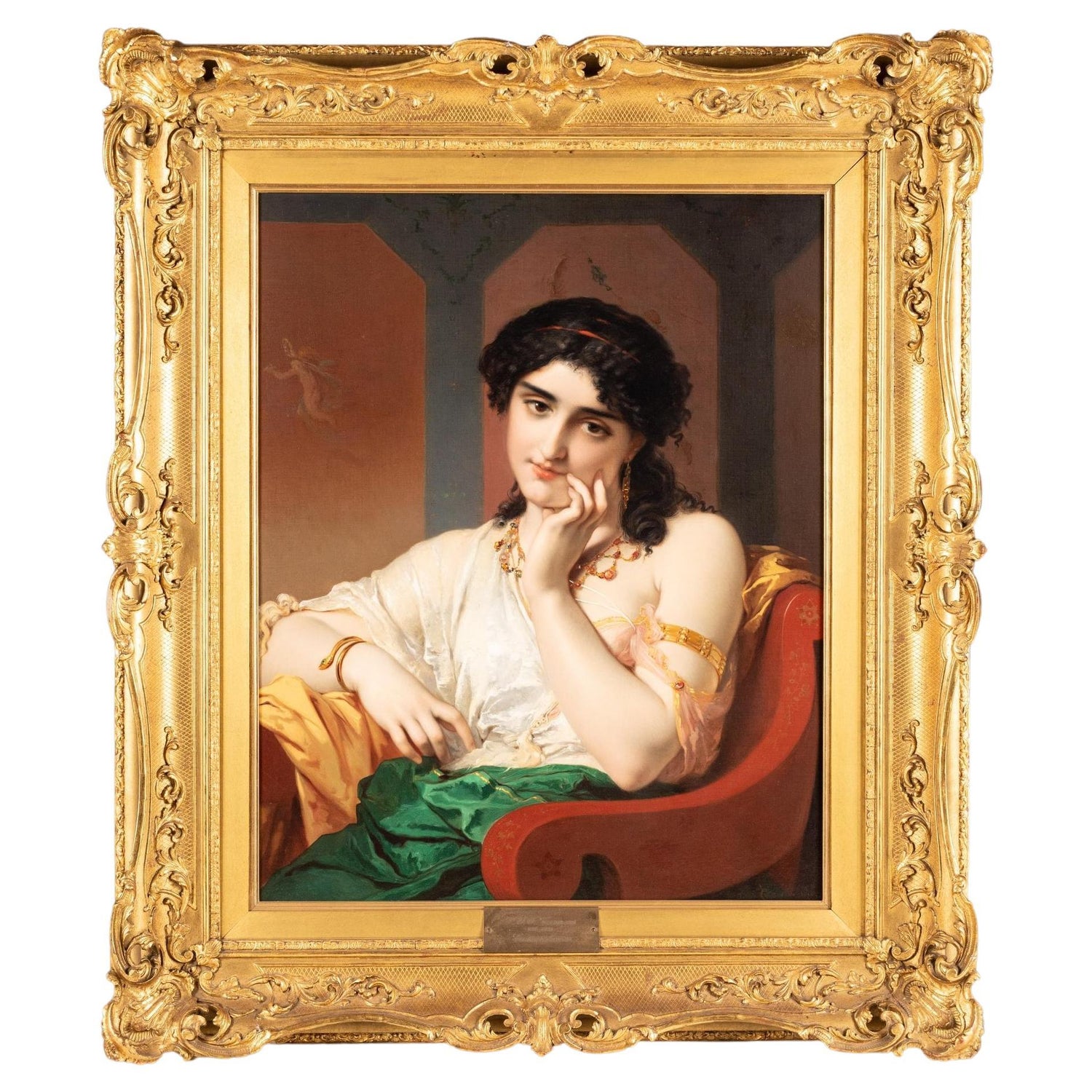This detailed portrait depicts a young, white woman with long, dark curly hair, elegantly styled with a red hair band and pulled back at the nape of her neck. She is seated in a richly engraved red wooden chair, her posture relaxed as she rests her head on her left hand with her fingers delicately touching her cheek, and her right arm comfortably positioned on the armrest. Her attire consists of a loose-fitting, off-white silk blouse that drapes over one shoulder, paired with a green skirt and adorned with ornate jewelry, including a snake-like bracelet on her wrist and a beaded necklace. The background features a brown wall with painted black columns, enhanced by ethereal images of angels or mythical creatures flying around an archway structure. The entire artwork is encased in an elaborate, thick golden frame with intricate details, resembling something one might find in a palace or museum, suggesting its historical and artistic significance.